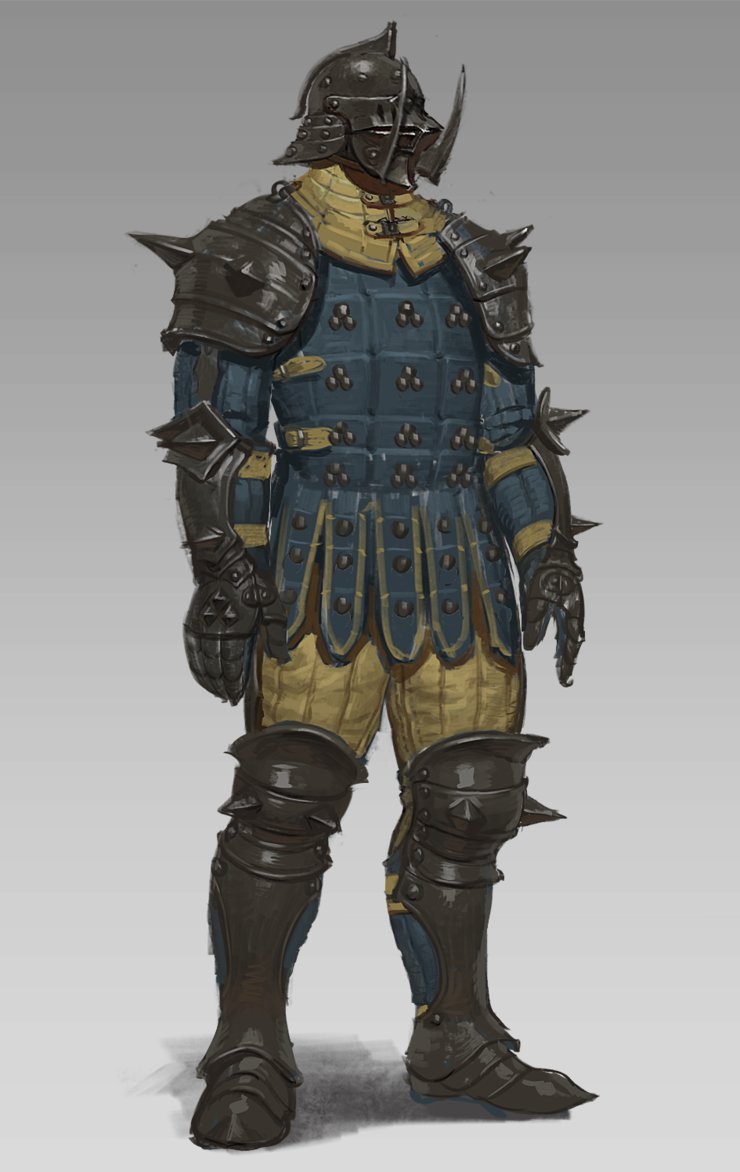This detailed concept art illustration features a muscular warrior clad in highly stylized medieval armor, likely inspired by European designs with samurai elements. The armor spans a gradient background that transitions from light gray at the bottom to darker gray at the top. The warrior is outfitted in dark gray metal armor, heavily adorned with spikes at the shoulders, elbows, knees, and wrists. His ornate helmet features protruding tusks, adding to the intimidating design.

The armor covers much of his body, except at the back of the legs, which remain partially exposed. His torso is protected by a blue chainmail-like material with intricate yellow detailing, including straps around the sleeves and chest, yellow outlining on cutout flaps around the pelvic area, and metal rivets studded along the chest and flaps. More yellow elements are visible in the form of a strap piece around the upper chest and neck, while his pants also carry beige and gold accents.

Complementing this detailed ensemble, the legs are further protected by dark gray metal armor down to the feet, replete with spikes. The character’s overall appearance, with its mix of blue and gold hues and medieval motifs, suggests a video game character or a fantastical warrior drawn from a blend of Asian and European martial traditions.